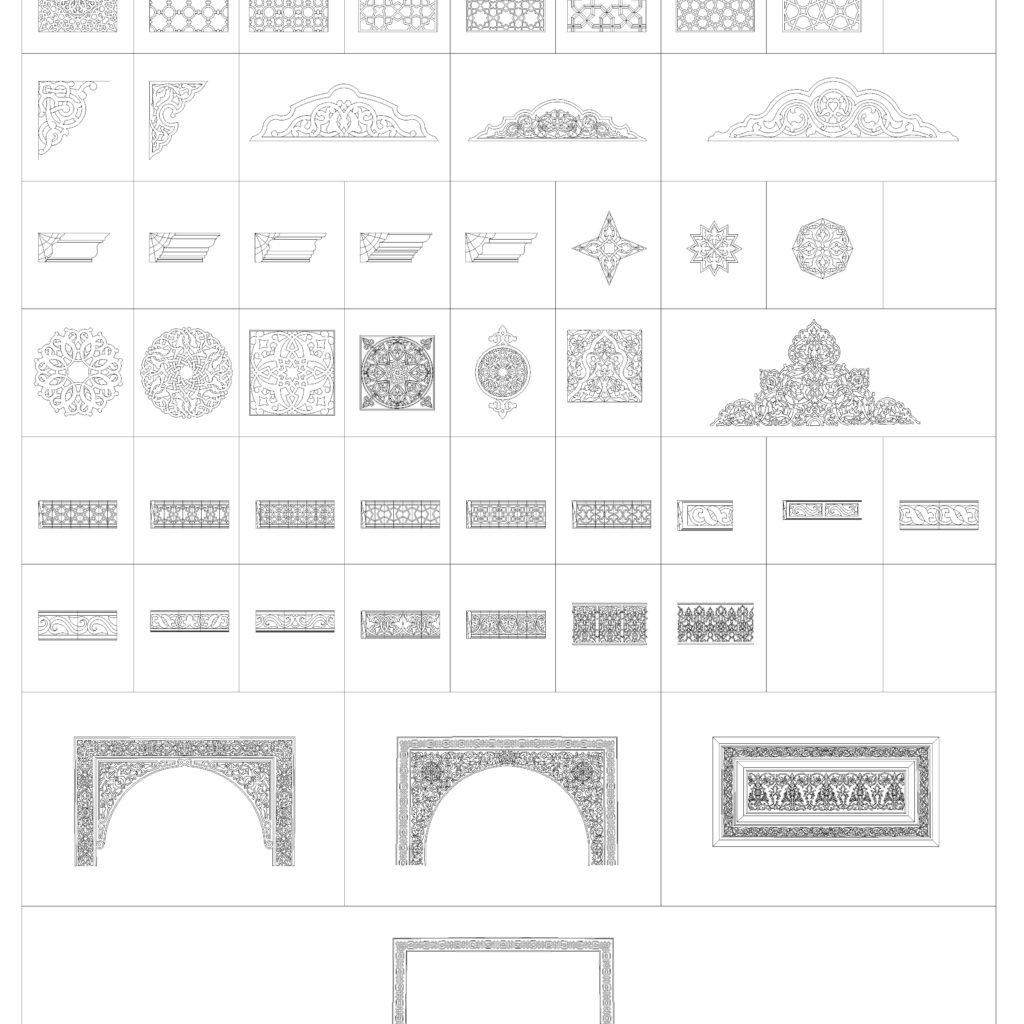The image depicts a collection of intricately detailed pencil sketches arranged in a grid format, consisting of various boxes containing unique stencil-like designs. Each box features distinct motifs that resemble architectural or decorative elements such as trim pieces, latticework, and emblems. The top row has eight small designs, including solid shapes, perforated pieces, and gate-like structures with cross patterns. Subsequent rows feature a variety of shapes, such as corner pieces, stars, sun-like symbols, and circles, some with additional elements protruding from them. Middle sections highlight rectangular and bold pieces, appearing as molding or wall décor. The bottom section showcases designs incorporating arches, creating squares with half-circle cut-outs, and a few larger rectangles. Overall, the black and white sketches serve as templates or guides for more detailed art or architectural work, demonstrating a broad spectrum of ornamental concepts.